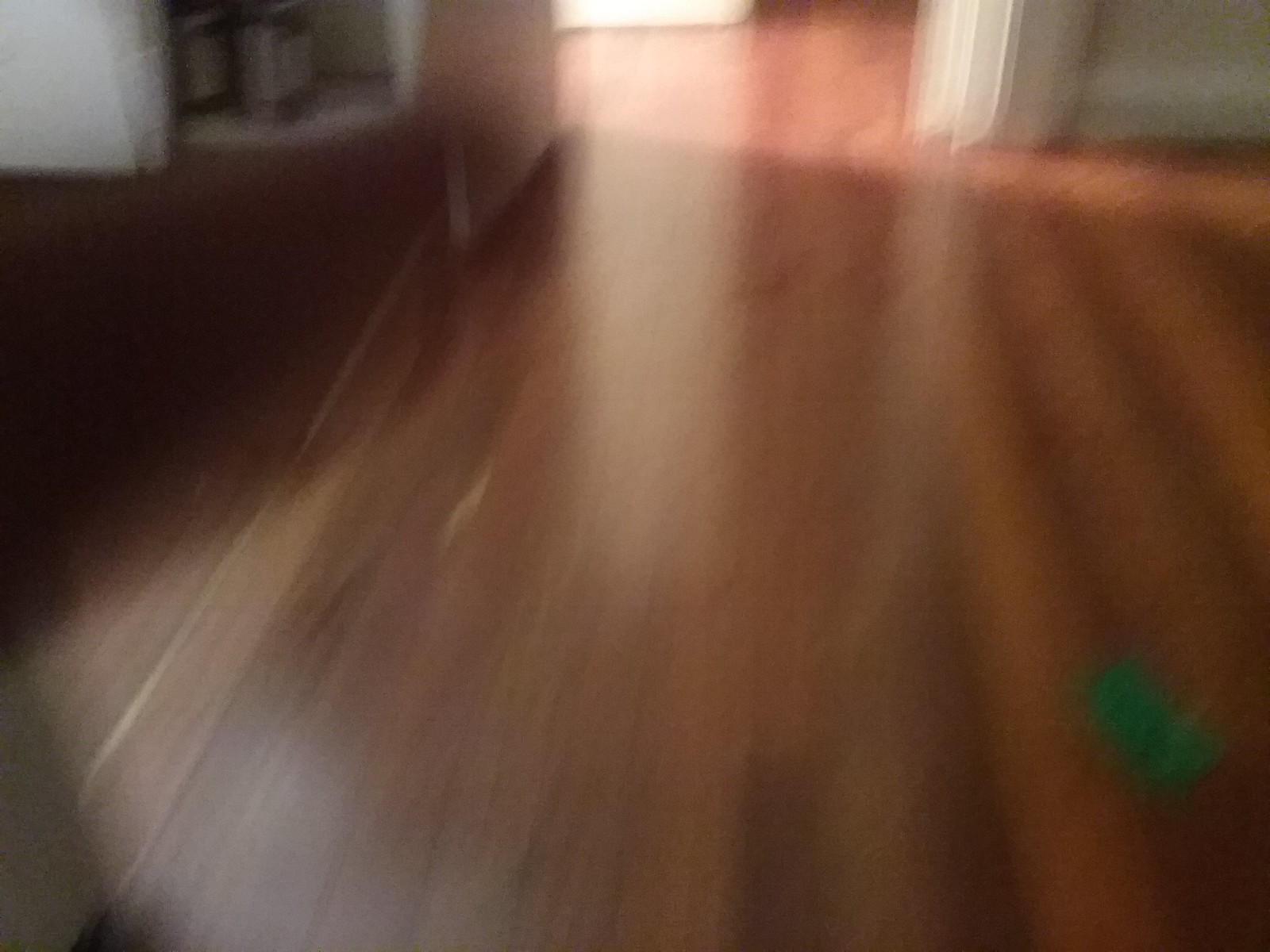The image depicts a bright and cheery room inside a house with an emphasis on the dark hardwood floor, featuring varying shades of brown. The photograph is blurry and lacks defined details, suggesting movement during capture. The room appears to be largely unfurnished or potentially not yet moved into, contributing to the cleanliness of the floor. A green object is visible on the lower part of the floor, but the blur prevents identification. Sunlight generously illuminates the space, enhancing the warm atmosphere. In the background, an open doorway leads to another room with similar flooring, flanked by a white wall on the left. On the right, an open cabinet, with a white interior, contains two dark bottles partially obscured by something white. Additionally, a closet in the image seems to contain various containers, possibly for paint. The overall impression is of a sparsely furnished, sunny room with clean, well-maintained hardwood flooring.